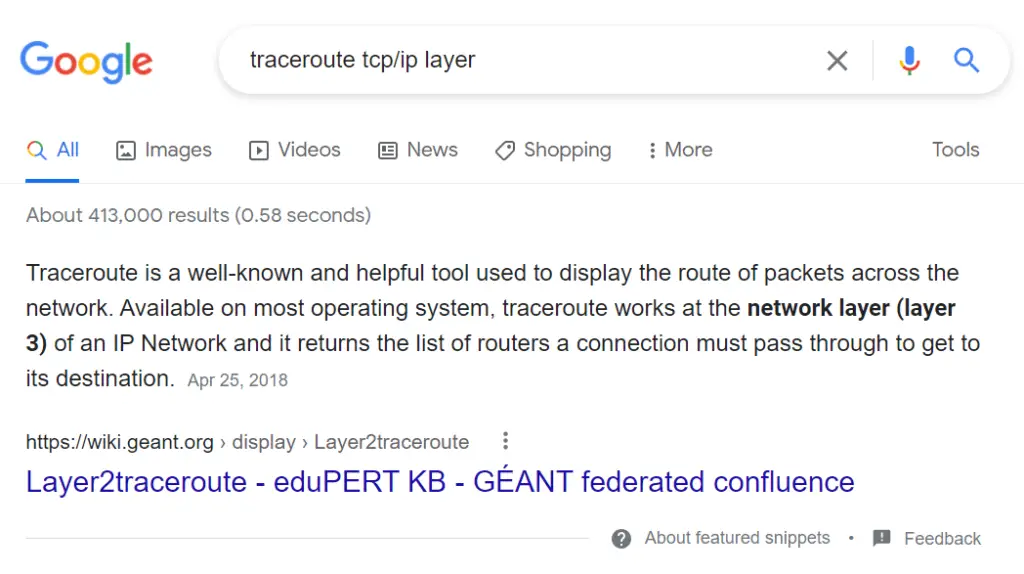This is a screenshot of a Google search result. The image features a white background, with the familiar Google logo displayed in the upper left corner. The logo consists of the word "Google" rendered in vibrant rainbow colors. Next to the logo is the search input field where the user has typed "trace route TCP/IP layer." This field also includes icons for clearing the text (small 'X'), voice input (microphone icon), and initiating a search (magnifying glass icon).

Below the search field is the Google menu bar, displaying options such as 'All', 'Images', 'Videos', 'News', 'Shopping', 'More', and 'Tools'. The 'All' option is currently selected. Beneath the menu bar, it is indicated that approximately 413,000 results were found in 0.58 seconds.

The top search result begins with the text in black font: "Trace route is a well-known and helpful tool used to display the route of packets across the network. Available on most operating systems, trace route works at the network layer, layer 3 of an IP network, and it returns the list of routers the connection must pass through to get to a destination." This entry is dated April 25th, 2018, shown in gray font, and the source of the information is a website with the URL "https://wiki.g.org".